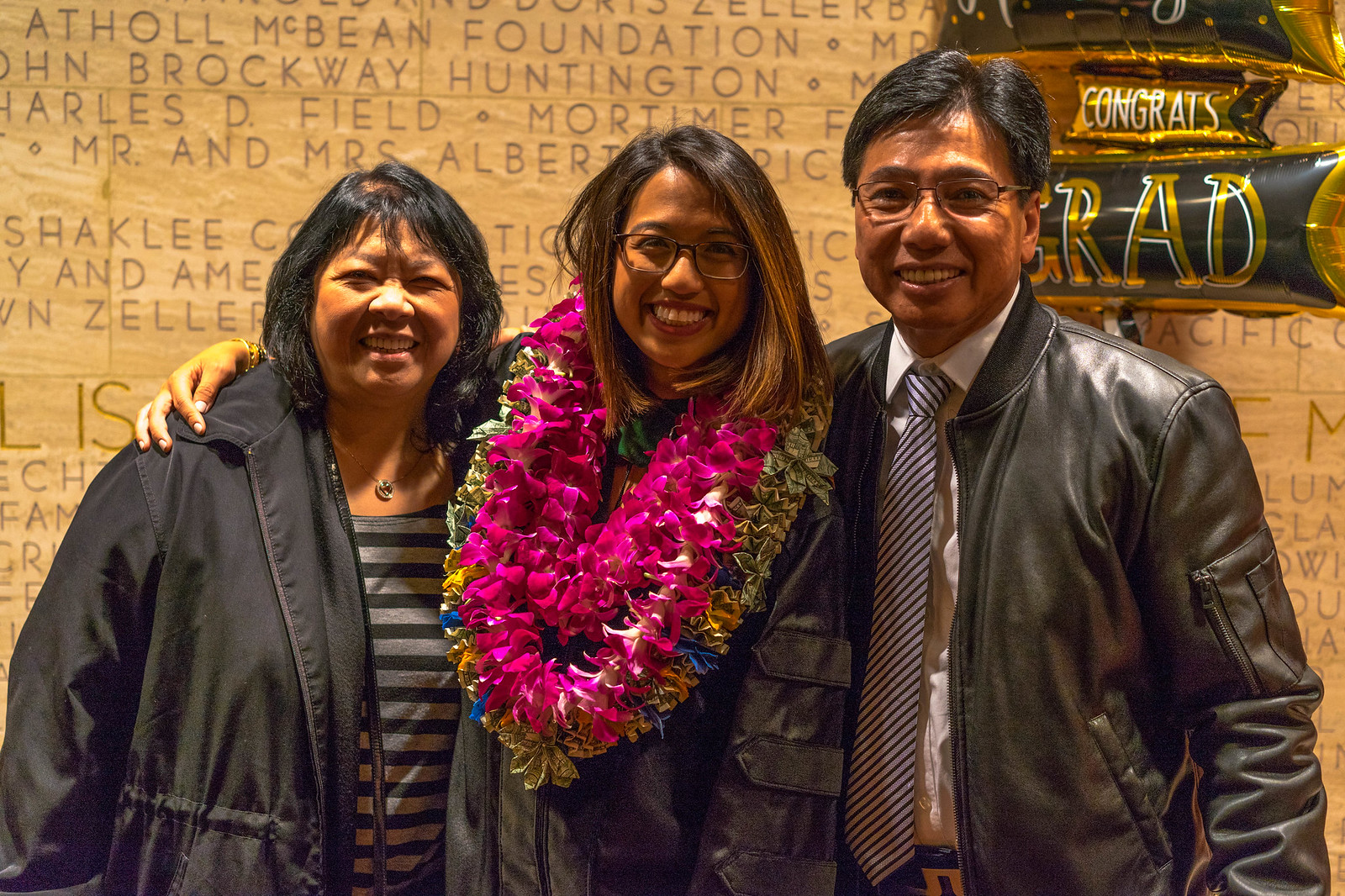This color photograph captures an exuberant family moment, with three people standing closely together, radiating happiness. The backdrop features celebratory balloons that spell out "Congrats, Grad," amidst a mix of other decorative elements. The subjects, likely Asian, consist of a woman on the left, a younger woman in the middle, and a middle-aged man on the right, suggesting a family dynamic, possibly the graduate and her parents. 

The woman on the left, with medium-length straight black hair, is dressed in a gray and black striped shirt, paired with a black jacket. The young woman in the center, presumed to be the graduate, is adorned with vibrant flower leis in pink, blue, and gold hues. She sports glasses and has medium-length dark hair with blonde highlights. Clad in a black jacket, she lovingly wraps her arm around the woman on her right. The man on the right, wearing a black leather jacket and wire-framed glasses, complements his look with a white dress shirt and a blue and white striped tie, a glimpse of a gold belt buckle visible at the bottom of the frame. Their genuine smiles and direct gaze into the camera capture the joy and pride of this significant milestone.